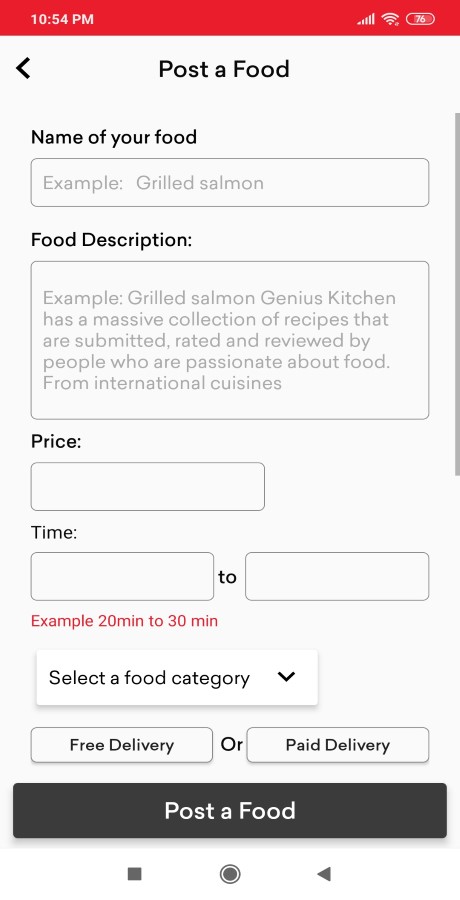The image is a screenshot taken from a cell phone displaying a food-related posting interface on a website or app dedicated to sharing and possibly selling food. The device time reads 10:54 PM, with the signal strength and battery level indicators visible in the top-right corner against a red bar. The main screen features a predominantly white background, centered with the heading "Post a Food" in bold black text.

Below that, there are several input fields for the user to fill out. The first field prompts the user to "Name Your Food," with an example provided: "Grilled Salmon." Next is the "Food Description" section, also accompanied by a sample description that reads: "Grilled salmon, Genius Kitchen has a massive collection of recipes that are submitted, rated, and reviewed by people who are passionate about food from various cuisines."

Further down, there are spaces for users to input the "Price" and "Time," with another example in red text indicating "20 minutes to 30 minutes." A drop-down menu allows users to "Select a Food Category." Additional options include choosing between "Free Delivery" or "Paid Delivery."

At the bottom of the screen, there is a prominent "Post a Food" button displayed on a gray bar with white text. The overall impression is that the site or app is likely a platform for posting, sharing, or selling food recipes or prepared dishes, though its exact nature remains unclear without further context.